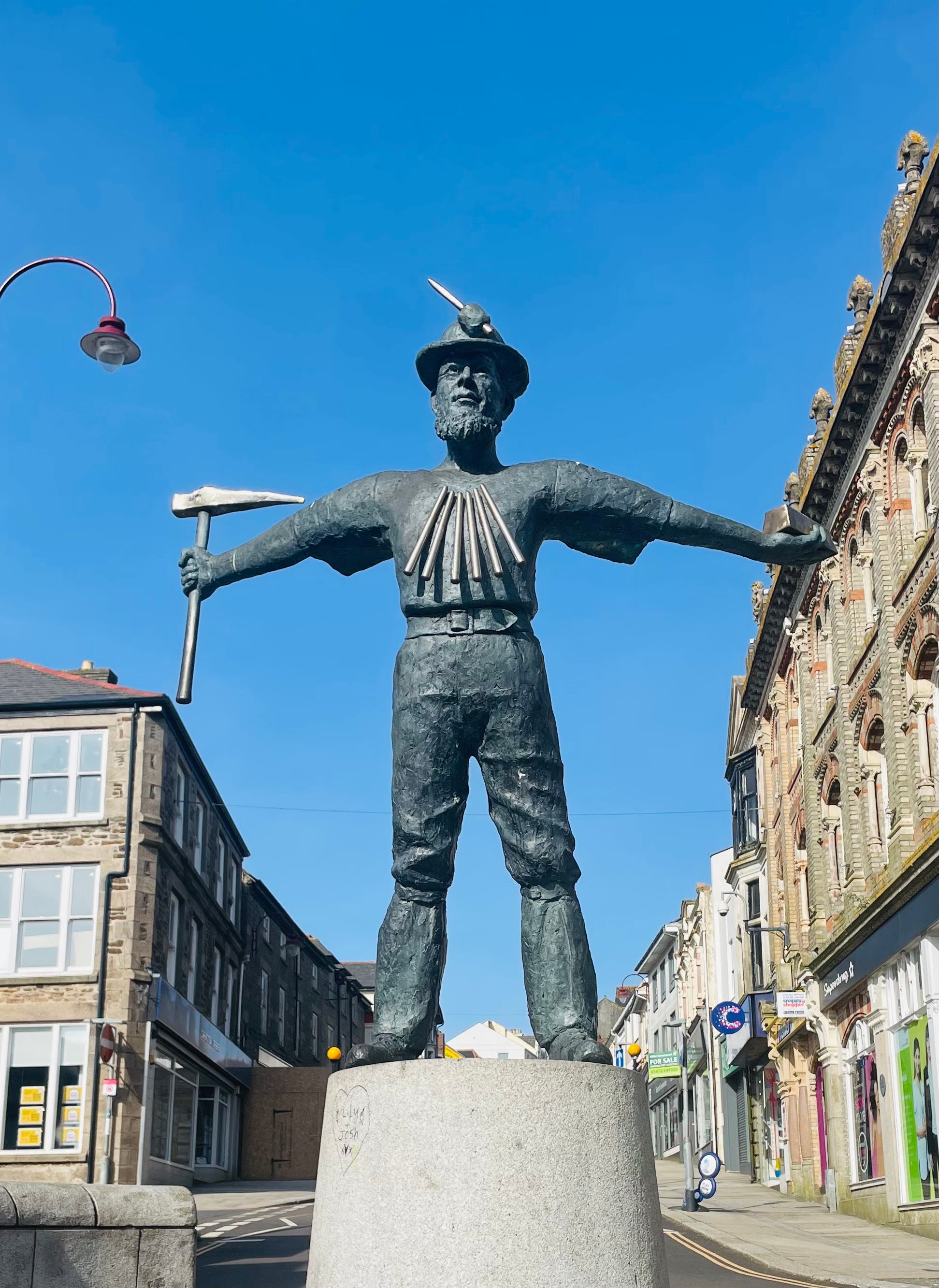The photograph, in a portrait layout, showcases a striking bronze statue of a man with his arms outstretched, centrally positioned within the frame. The man, resembling a Paul Bunyan-esque figure, stands on a tall cylindrical concrete base, which has a carved heart and two names etched into it. In his right hand, he grasps a large hammer with a pick, while his left hand holds a metal ingot. Adorning his head is a round-rimmed hat with a metal spike protruding through a ball at the top, suggesting a miner or construction worker. Five cylindrical, vertical-shaped metal pieces hang from his shirt, and he sports a beard, a belt, pants, and boots, all crafted from a dark, charcoal-colored metal. The backdrop of the image reveals a narrow asphalt road flanked by multi-storied townhomes, contrasting against a blue sky. Notably, the scene is devoid of traffic and people, highlighting the statue’s solitary prominence.